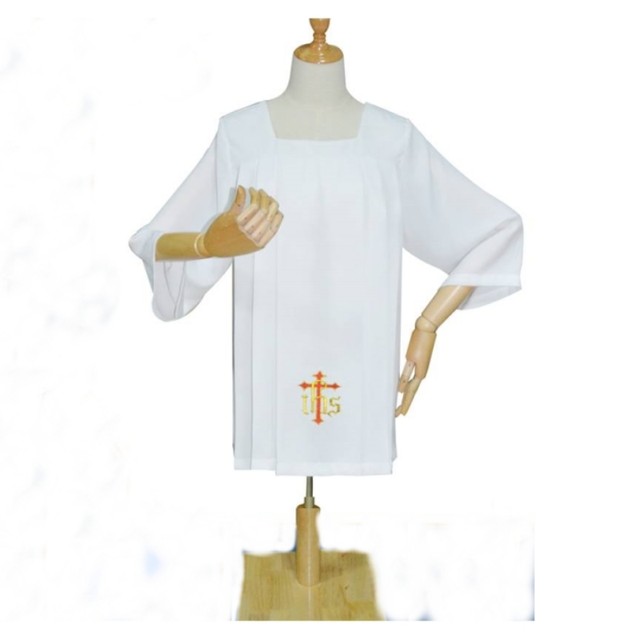This is a color photo featuring a headless mannequin with wooden, foldable arms on a simple wooden stand. The mannequin is dressed in a white religious tunic, possibly a Catholic choir robe, with three-quarter length sleeves and a square neckline. The robe is entirely white except for the bottom, which bears a prominent red cross adorned with gold decorative elements and the letters "LHS" embroidered in gold. One of the mannequin's hands is positioned on its hip, while the other is placed in front of its body. The background of the image is a solid white, highlighting the tunic and its intricate details.